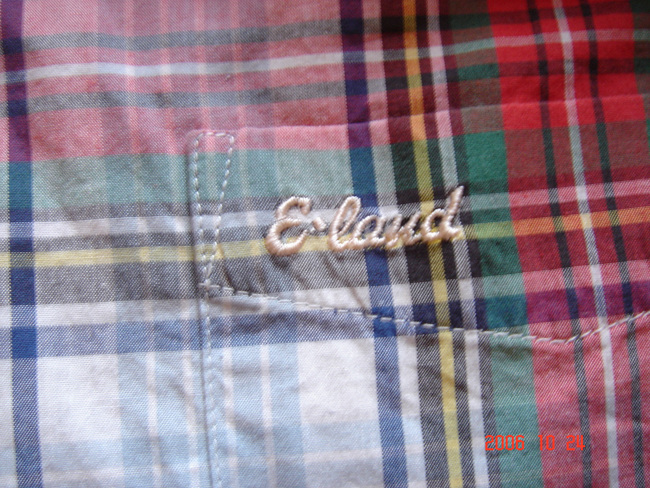This detailed photograph captures a plaid article of clothing, with a date stamp in red at the bottom reading "2006-10-24." The fabric appears somewhat washed out, with a color palette that includes shades of green, white, black, red, yellow, gold, blue, and light blue. The focal point of the image is a pocket, highlighted by visible white stitching, including some off-white embroidered letters and horizontal stitches that contribute to the worn, faded look of the pocket area. To the left of the image, near the date stamp, the plaid pattern prominently features green, red, and black. On the right side, the pattern includes an array of colors like black, white, green, yellow, blue, and light blue. The photograph is of excellent quality, vividly capturing the details of the fabric and stitching.